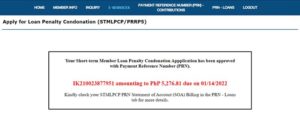The screenshot depicts a largely unreadable image featuring a user interface. At the top, there is a blue bar containing a series of words or instructions that are not clearly distinguishable. Directly below the blue bar, there is black text which appears to say "apply for loan penalty" or something similar. The remainder of the screen consists of a predominantly white section containing a series of small, indeterminate boxes. Within this white section, there is a long enclosed square with various lines of text. The text includes a longer sentence in black, a shorter sentence in red, and very tiny, almost unreadable font beneath it. The overall layout and text content suggest it might be related to a loan application or financial form, but the exact details remain unclear due to the illegibility of the image.